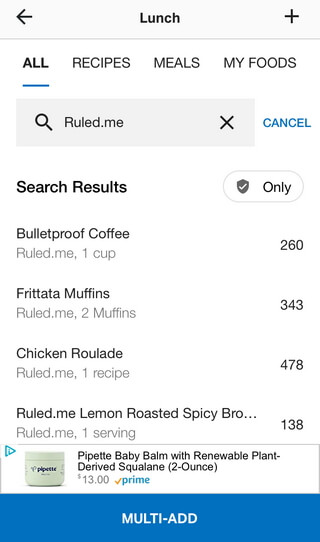The image shows a screenshot of a smartphone application designed for tracking recipes and food intake. The interface features a top banner in an off-white color, with a back arrow icon on the top left corner and a plus icon on the top right corner, presumably for adding new food items. Centrally located in the banner is the word "Lunch." 

Below this banner, there are four tabs labeled "All," "Recipes," "Meals," and "My Foods," with the "All" tab currently selected. Directly below these tabs is a search bar displaying the text "ruled.me," indicating a recent search. 

The search results are listed as follows:
1. Bulletproof Coffee from ruled.me, one cup, 260 calories
2. Frittata Muffins from ruled.me, two muffins, 343 calories
3. Chicken Roulade from ruled.me, one recipe, 478 calories
4. Lemon Roasted Spicy [word cut off] from ruled.me, one serving, 138 calories

An advertisement follows the search results, promoting a product called Pipette Baby Balm with renewable plant-derived squalane, priced at $13 for a 2-ounce container, available through Amazon Prime. 

Overall, the app appears to be a comprehensive tool for logging meals and their nutritional content, possibly including calories or carbohydrates.